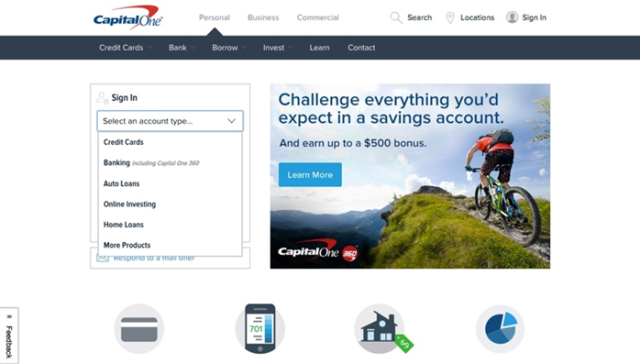This is a screenshot of the Capital One website homepage. The top section features a white banner with the Capital One logo and several clickable options. These include "Personal" (currently selected), "Business," and "Commercial." Below this banner, there's a navy sub-banner providing a dropdown menu with options for "Credit Cards," "Bank," "Borrow," "Invest," "Learn," and "Contact." To the right of the navy sub-banner, there are "Search," "Locations," and "Sign-in" buttons.

On the left-hand side of the page is a sign-in box for personal accounts. The "Select an account type" dropdown menu is open, listing different account types: "Credit Cards," "Banking," "Auto Loans," "Online Investing," "Home Loans," and "More Products." This list partially obscures the username and password fields, suggesting their presence underneath.

To the right of the sign-in box, there is an advertisement for Capital One, featuring an image of a mountain biker ascending a mountain. The ad text reads, "Challenge everything you'd expect in a savings account and earn up to a $500 bonus. Learn more."

Near the bottom of the page, four icons serve as quick navigation buttons: a credit card icon, a credit score icon, a mortgage icon, and a pie chart icon. Additionally, a small feedback tab is visible in the bottom left corner of the screen.